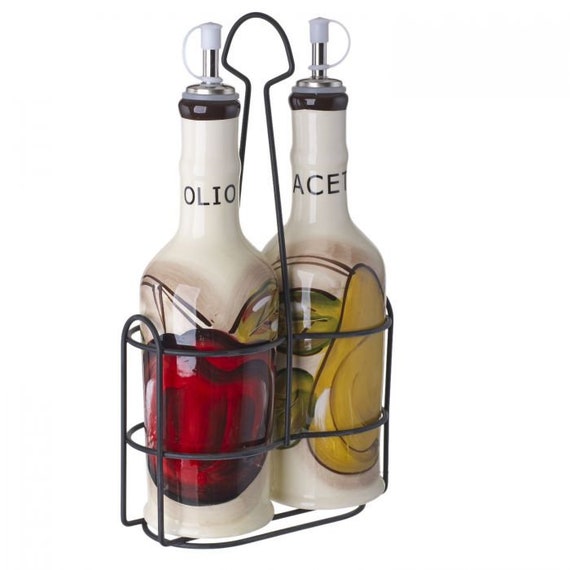The image depicts a cruet set designed for a restaurant table, consisting of two white ceramic bottles held by a black metal wire holder with a central handle for easy transport. The bottle on the left is labeled "OLIO" and features a detailed illustration of a red pepper with a black outline and green stem, fitted with a stopper for dispensing oil. The bottle on the right has partial lettering that reads "A-C-E-T" and showcases a painted green avocado and possibly another green fruit, also equipped with a stopper. The backdrop of the image is plain white, highlighting the cruet set's design and functionality for storing condiments like oil and vinegar.